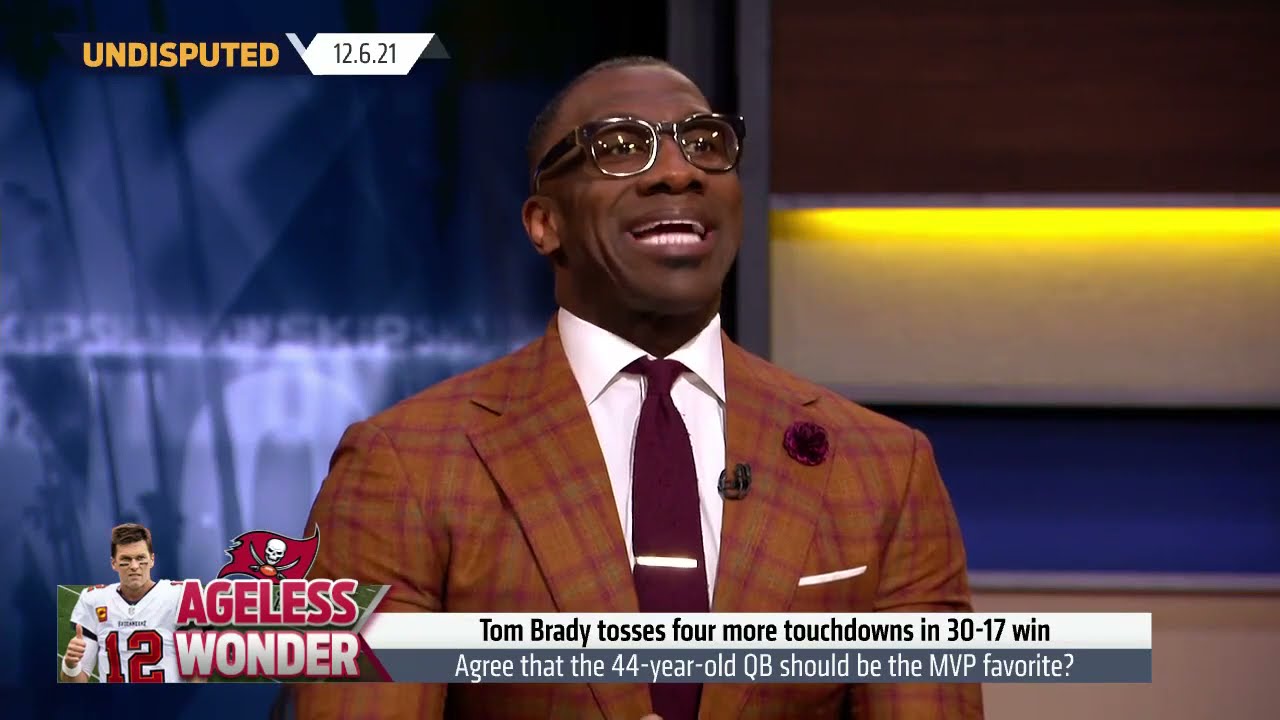The image is a still from the sports TV show "Undisputed," featuring a well-dressed African-American sportscaster wearing glasses. He is adorned with a distinctive reddish-brown plaid suit jacket over a white collared shirt and a burgundy tie secured with a tie clip. The man, who appears to be mid-sentence with his mouth open and a smile, showing shiny pearly white teeth, faces forward with a slight orientation to the right. The background is dark blue, and in the upper left corner of the image, the show's title, "Undisputed," is displayed in capitalized yellow letters along with the date, "12.6.21," in a white shape with navy text. Beneath the sportscaster, there is a smaller image of Tom Brady in his Tampa Bay Buccaneers jersey, accompanied by the text "Ageless Wonder." Additional text reads, "Tom Brady tosses four more touchdowns in 30-17 win. Agree that the 44-year-old QB should be the MVP favorite?" The detailed setup and enthusiastic demeanor of the sportscaster suggest he is likely discussing Tom Brady's recent performance and his MVP candidacy.